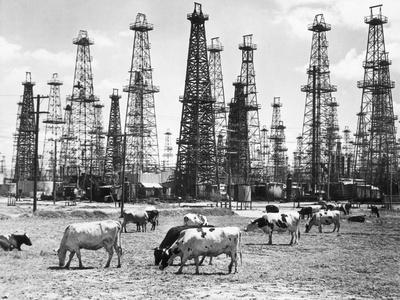This is a small rectangular black-and-white photograph depicting a herd of approximately 15 cattle grazing in a field with patches of rare dirt and edible plants. The cattle vary in color, including white, black, and spotted varieties, and most have their heads down as they graze. In the background, a large number of towering oil wells dominate the landscape, with their metallic rigging and vertical tubes prominently visible. The tallest towers are positioned toward the front, decreasing in size as they recede into the distance. Additionally, telephone poles with wires are visible along the left side of the image. The sky appears cloudy, adding a serene backdrop to the scene.